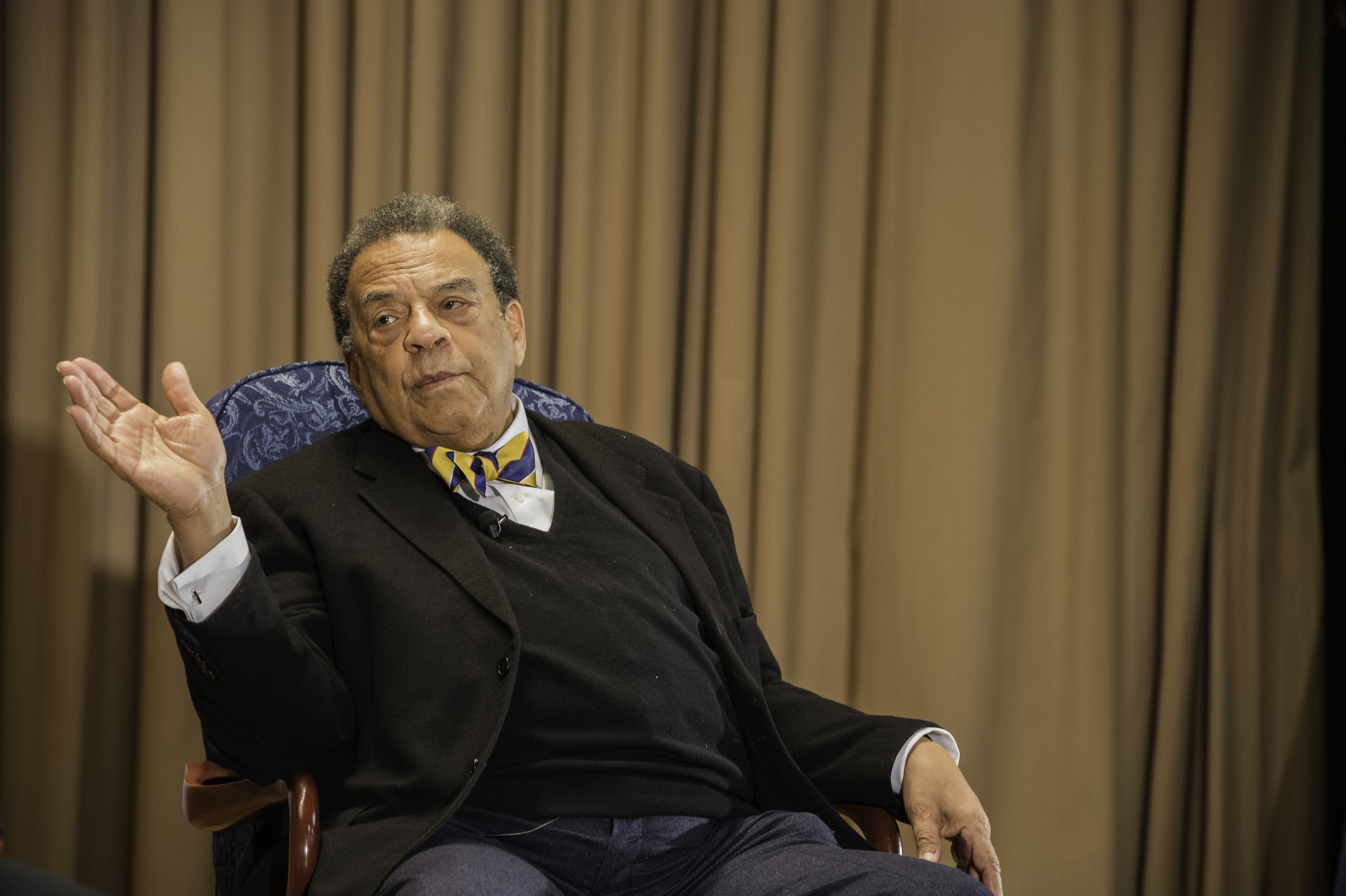The image depicts an indoor event, potentially a speaking engagement, featuring an older man seated in a blue, cushioned chair with wooden armrests and a white swirling pattern. The background is a continuous beige curtain stretching from left to right. The man, dressed in a black blazer over a black sweater vest and a white button-down shirt, sports a distinctive yellow and purple striped bow tie. He has grayish hair and a serious expression, suggesting he is deep in conversation or explaining something. A microphone is pinned to his sweater, and he sits with his left elbow resting on the chair’s armrest, his right arm slightly raised with the palm facing outward as if gesturing thoughtfully.